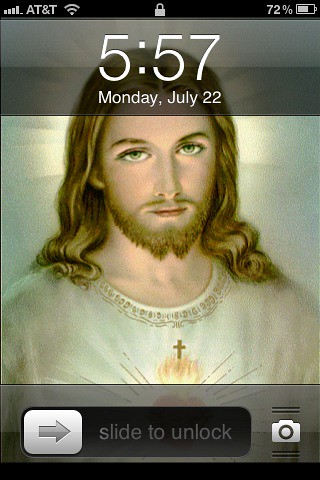The screenshot appears to be taken from an older model iPhone, likely around 2010. At the top of the screen, the status bar shows AT&T as the service provider, with the service bars, Wi-Fi signal symbol, a lock icon, and a battery icon indicating 72% charge. The time is displayed prominently in white text as 5:57, just above the date, Monday, July 22nd. The wallpaper features a well-known depiction of Jesus Christ, wearing a white tunic with gold embroidery, a small cross on his chest, and a flaming heart symbol. Jesus is portrayed with flowing light brown hair, gentle green-blue eyes, and a small mustache and beard, looking forward serenely. Below the wallpaper image, there is a "slide to unlock" bar with an arrow pointing to the right and a small camera icon that allows quick access to the camera.